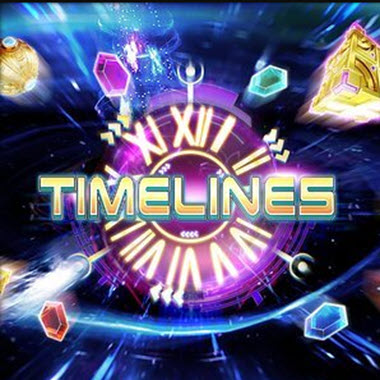The image is a detailed, vibrant graphic reminiscent of a video game screenshot. Central to the composition is a glowing magenta clock with gold Roman numerals ranging from I to XII. The word "timelines" is prominently displayed in large yellow-gold text with a greenish outline in the center of the clock. Surrounding the clock are various colorful gemstones flying outward—purple, green, blue, and red—each leaving a trailing blur that adds to the overall dynamic feel. The background is a dark, starry, night sky, adding a magical and space-like ambiance to the scene. Notably, a golden cube is present in the top right corner, while a golden sphere, resembling a Christmas ornament, occupies the top left. Both items appear to be in motion, complementing the twirling effect of the gemstones, enhancing the sense of animation and excitement in the image.